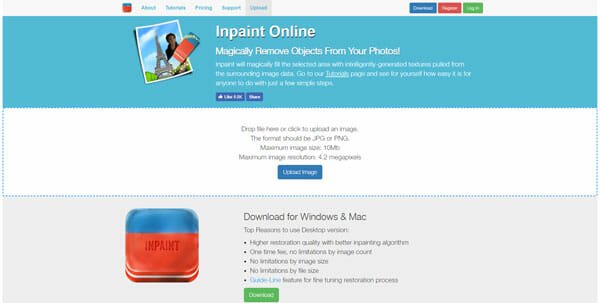The screenshot depicts a colorful and detailed landscape-format webpage for a company specializing in photo editing, named "InPaint Online." This company offers a service that allows users to magically remove objects from their photos. The headline prominently displayed at the top of the screen reads, "InPaint Online: Magically Remove Objects from Your Photos!" Below this, an illustrative image demonstrates the software's capability. It shows a person standing in front of the Eiffel Tower, with an eraser tool seemingly removing the individual from the scene. 

In the central section of the webpage, users are prompted to either drop an image or click to upload a photo for editing, suggesting that the primary function of the site is to allow users to manipulate their images directly online. The fee structure, if any, is not visible in this screenshot. 

Beneath this upload section, there's a panel titled "Download for Windows Mac," which lists several compelling reasons to opt for the desktop version of the software. At the top of the page are multiple tabs, though the text is not entirely clear. The user appears to be on the "Upload" tab, as suggested by the context of the visible section for uploading images.

This detailed layout clearly indicates that the service is designed for user-friendly photo editing, offering both online and desktop solutions.